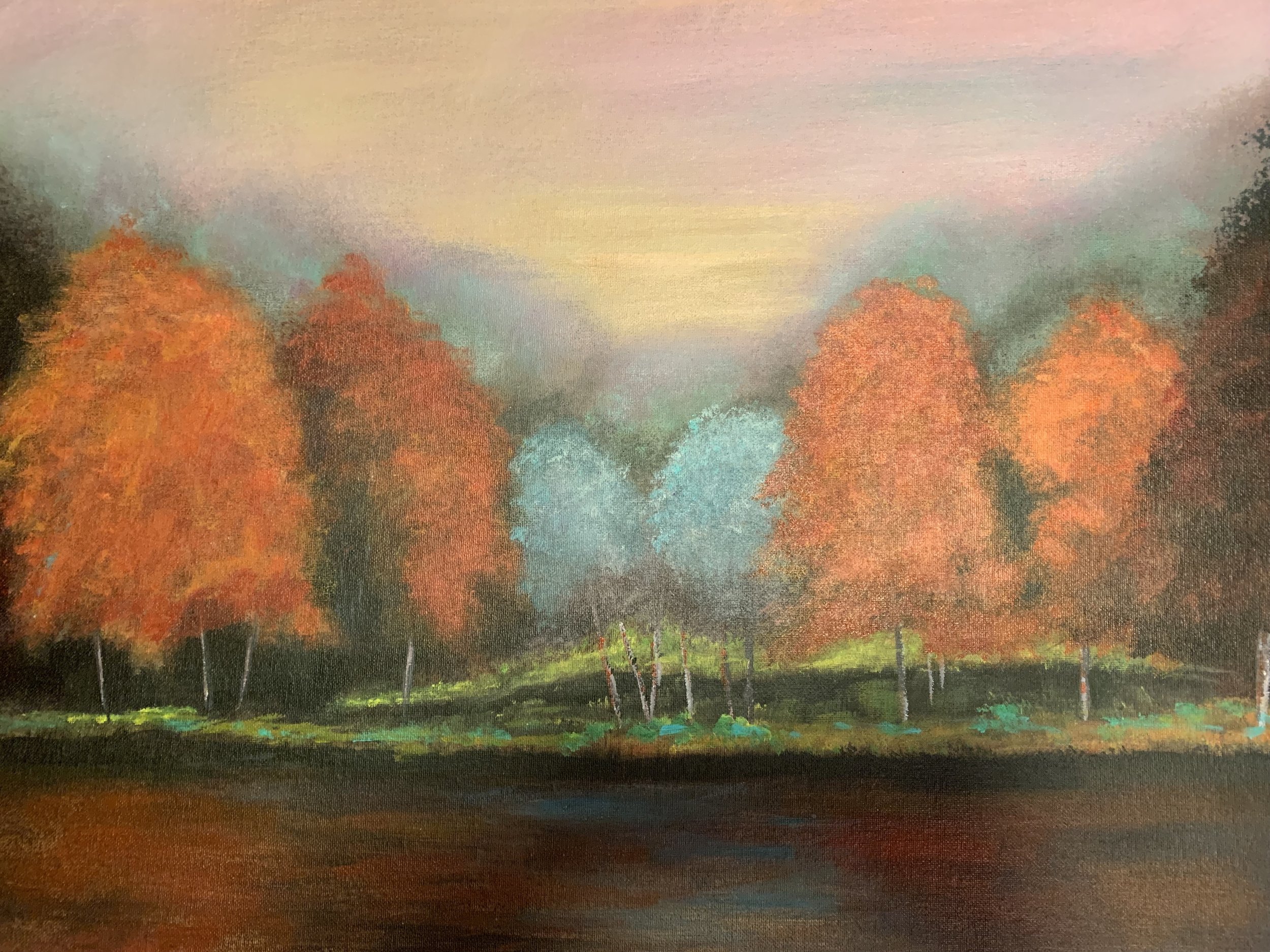The painting depicts a serene nature scene featuring a dark, murky lake or stream in the foreground. Beyond the water lies a grassy field adorned with blue bushes, creating a sense of natural beauty. The trees along the bank exhibit a blend of oranges, reds, and some dark brown hues on the right side, suggesting an autumn setting. The foliage, though indistinct and splotched, clearly identifies the forms as trees, with some central ones displaying different tones, possibly greenish-blue. Above the scene, the sky transitions from a warm yellow to a rich red, hinting at a sunset, with small white clouds clustered in the top right corner. The overall style of the painting is blurred and impressionistic, lacking fine detail or a visible artist's signature. Despite the indistinct style, the painting captures the essence of a tranquil, autumnal landscape.